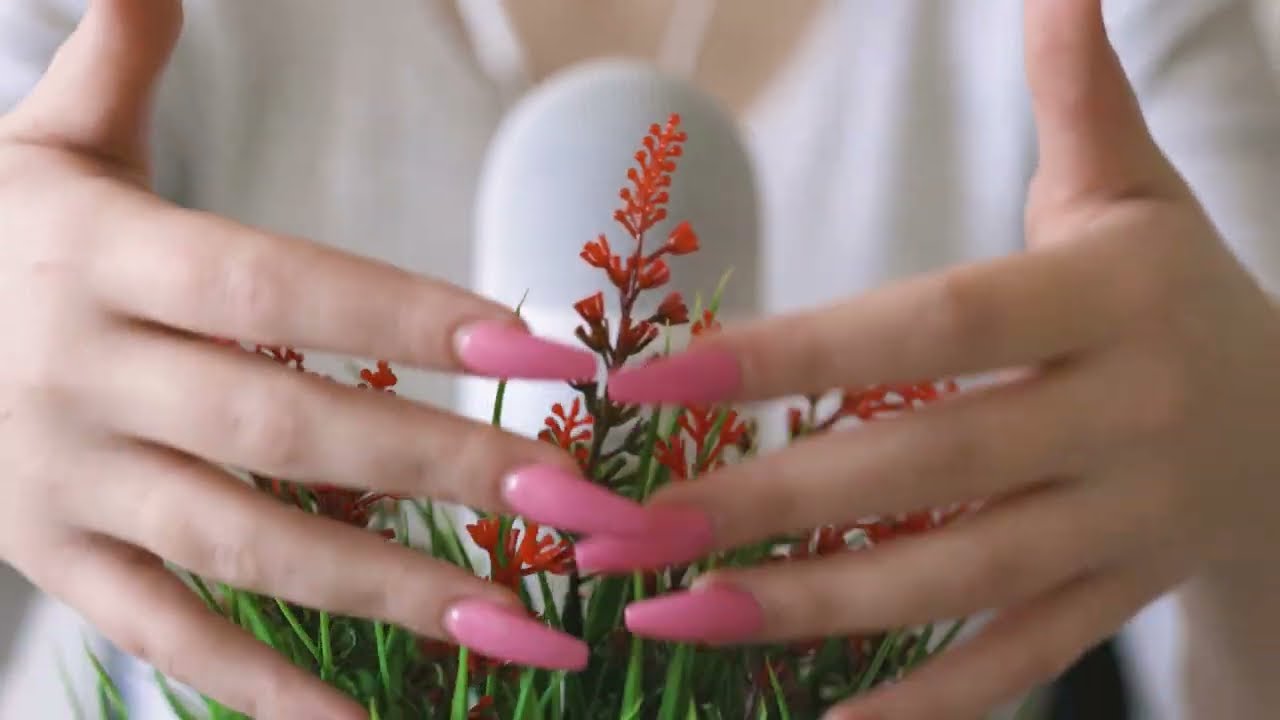In the center of the image, a woman's hands, adorned with long, bubblegum pink fingernails, are gently caressing a small green plant with delicate red flowers. The hands are splayed out, allowing us to see the vibrant little blooms through the fingers. The woman's fair skin contrasts with her bright nails and the lush greenery she is touching. Her thumbs are positioned upward, creating a framing effect around the flowers. Behind the plant, we can see her blurred figure dressed in a white blouse, adding a subtle backdrop to the scene. A white, round object that resembles a microphone is positioned in front of her, adding an intriguing element to the composition. The colors throughout the image—green leaves, red flowers, white blouse, and pink fingernails—create a vibrant yet soft visual palette. The setting appears ambiguous, potentially indoors or outdoors, with no text present to provide further context.